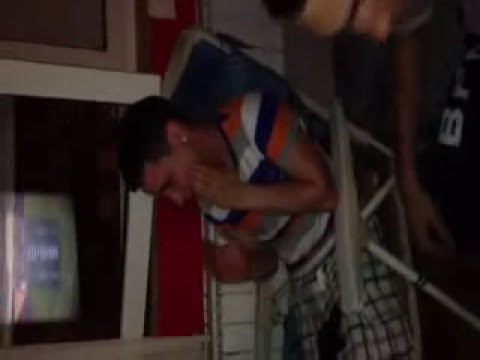The image depicts a boy with short, dark hair and an earring in his left ear, sitting in a beach chair, oriented 90 degrees counterclockwise. He is wearing a striped shirt featuring white, blue, orange, and tan colors, along with plaid shorts in shades of gray, white, and black. His left arm is bent at the elbow, with his hand resting on his cheek in a pensive manner. Beside him, to the side of his face and slightly obscured, there's another individual whose features are less visible. This second person is wearing attire with the letters "BR" noticeable and possibly a black T-shirt. In the background, there is a brick-lined red wall adorned with a framed object, potentially a television or computer screen, which is black inside the white frame.